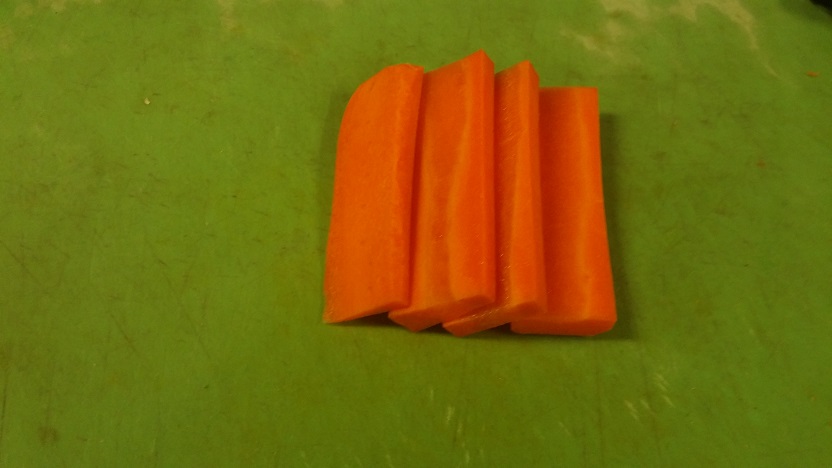The image depicts four uniformly cut carrot slices laid out on a dark celery green background. The vibrant, bright orange color of the carrots suggests they are fresh and safe to eat. Each carrot slice is approximately three to five inches long and about a quarter of an inch thick, with one slice being slightly thinner than the others. The slices are arranged neatly in the center of the green rectangle, potentially forming an accordion-like layer, indicating precision in their preparation. The green background appears to have been used for slicing and chopping, judging by the cut marks, though the exact material remains unclear.